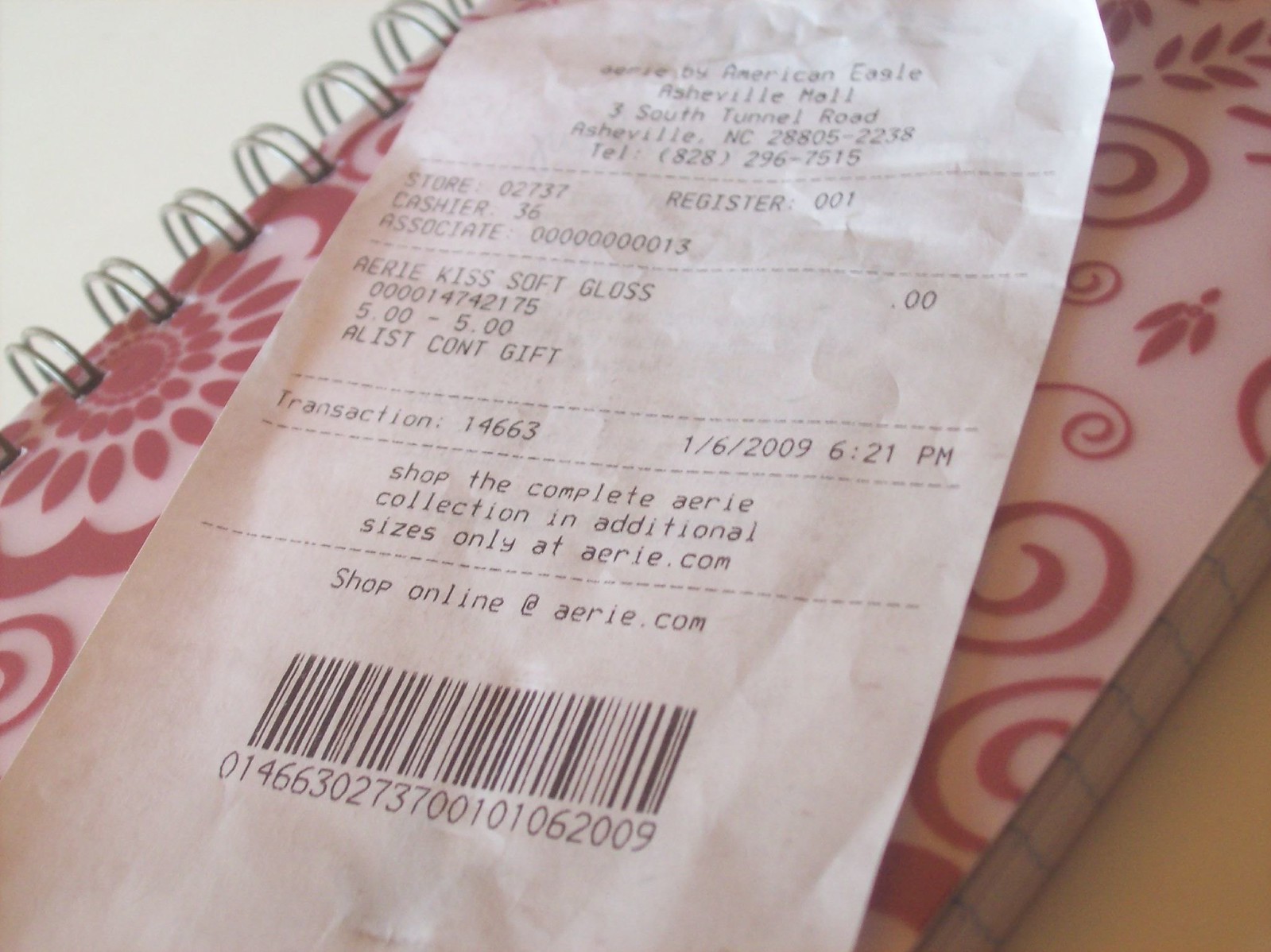This image displays a detailed receipt from an American Eagle store located at the Asheville Mall, specifically at 3 South Tunnel Road, Asheville, North Carolina, 28805. The store's contact number is (828) 296-7515. The receipt indicates transactions made at store location 02737, using register 001, handled by cashier number 36. The associate involved in the purchase is identified by a numerical code ending in 13. The item purchased was an Aerie Kiss Soft Gloss.